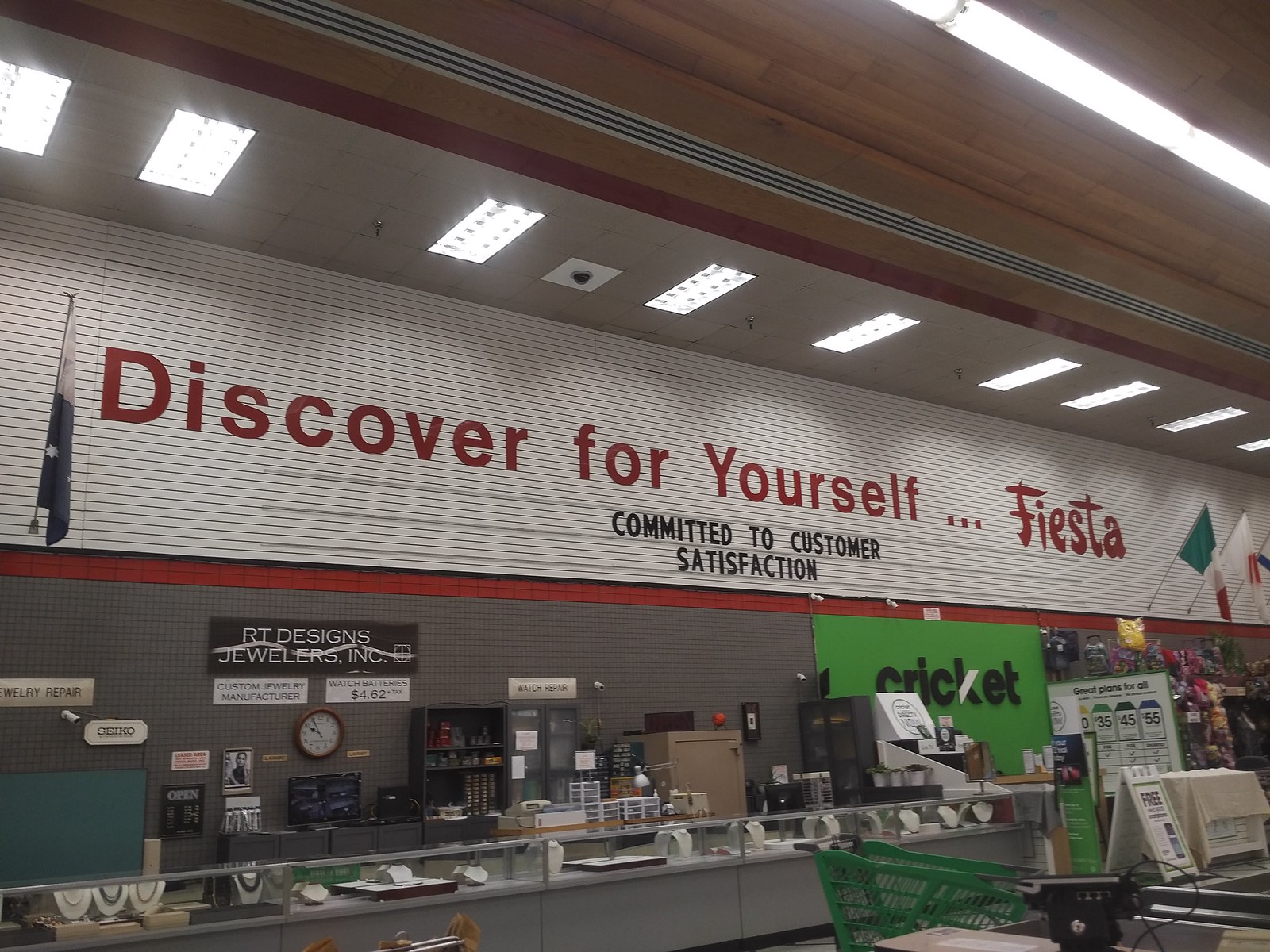The photo depicts the interior of a jeweler's store, as indicated by the signage. At the top of the image, there are fluorescent lights and a light wood ceiling. Below that, a wall painted white has red text proclaiming "Discover for yourself Fiesta" and black text that reads "Committed to customer satisfaction." 

Beneath this, on a gray wall with a red horizontal stripe, there's a sign in white and black letters stating "R.T. Designs Jewelers Inc." Directly below this sign, a wooden clock is visible. The wall also features several photographs and an "Open" sign.

In the lower section of the image, there is a glass jewelry display case with a gray bottom, showcasing jewelry on white displays. Adjacent to this, on a green section of the wall, the word "cricket" is written in black, accompanied by signage for Cricket Wireless. Additionally, the upper part of the "Fiesta" section of the wall is adorned with what appears to be a Mexican flag.